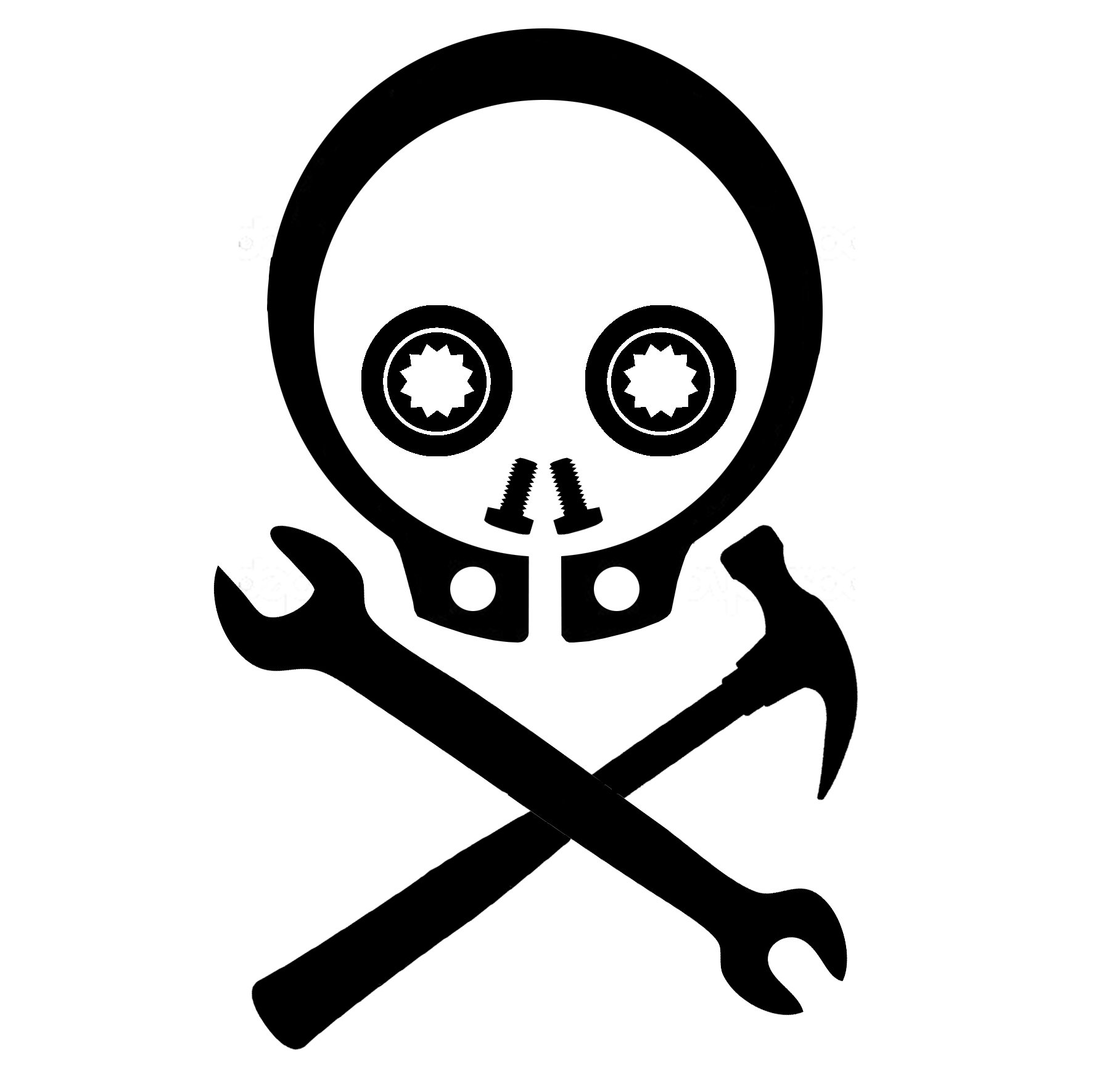The image displays a digital graphic, predominantly in black and white, embodying a stylized, menacing skull. The 'face' of the skull is a black-rimmed white circle with two large, circular eyes characterized by internal jagged wheel patterns outlined in white. The nose is represented by two inverted screw heads forming a low shape, and the mouth appears as two small holes. Below the skull, a hammer and a wrench are crossed in a manner reminiscent of the crossbones beneath a pirate skull. Absent of any text, the graphic maintains a clean, monochromatic aesthetic and could be representative of a logo, possibly for a home improvement company or as a stock image, evoking simplicity and technicality.